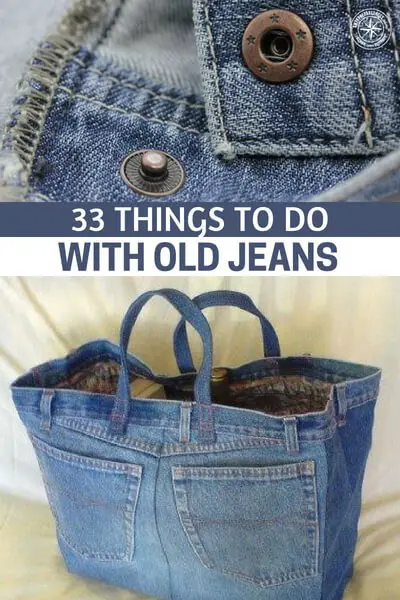The image features two detailed photographs showcasing creative uses for denim products. The top photograph is a close-up of metal slap buttons attached to a small section of denim fabric, and the image is tall and rectangular. Below it, prominently in the center, text reads "33 things to do with old jeans," with the phrase "33 things to do" in white on a blue background, and "with old jeans" in blue on a white background. The bottom photograph displays a rectangular denim bag prominently featuring two large front pockets. The bag, highlighted against a white sheet background, showcases three belt loops on the front top edge and one on the right side. It has a pair of handles, and inside the bag, the lining is brownish-black. A bottle of liquid sits in one of the pockets, with a yellow box positioned next to it. The overall theme of the image centers around innovative and practical repurposing of old denim garments.